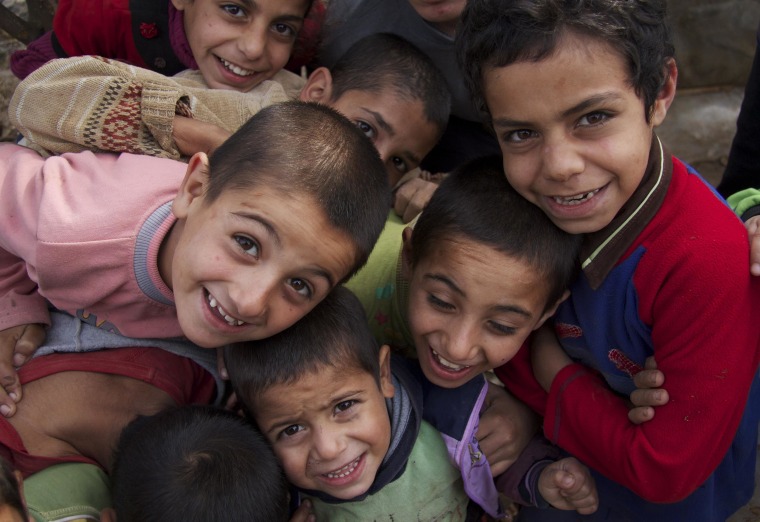The image features a group of eight young children, likely aged between two and four years old. They have short, dark brown hair and are mostly smiling, though some smiles appear more natural than others. The children, who may be from a Middle Eastern, Asian, South American, or possibly island region, are all wearing long-sleeved shirts in various colors including red, blue, green, lime green, and pink, although one child has a shirt with both blue and red sleeves. Their clothing appears reminiscent of styles from the 70s or 80s. In terms of composition, five children's complete faces are visible, one child's face is partly seen, another's back of the head is visible, and only a part of a neck and dark blue shirt of the last child can be seen. The child on the far right is notably smiling with arms folded, and another child in a lime green top is looking up with a slight smile. The background has a brownish hue, adding to the nostalgic feel of the photo. The children’s expressions convey a mix of joy and subdued contentment, offering a poignant glimpse into their lives.